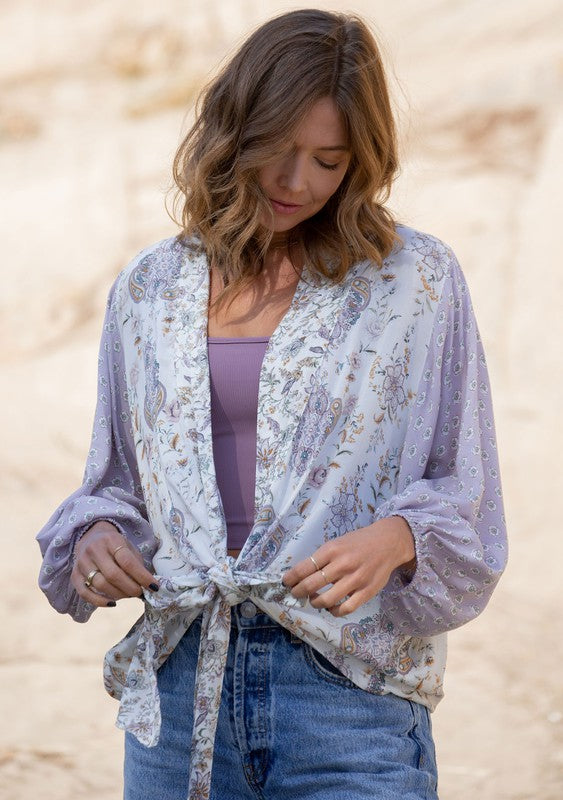In this portrait-oriented photo, a woman is captured from her thighs up, set against a blurred, tan-colored backdrop. She appears to be in her 40s or 50s, with mid-length, wavy, dark blonde to strawberry brown hair that falls just below her shoulders. Her eyes and head are inclined downwards, focusing on her hands, which boast dark painted nails and silver rings. She is adorned in a flowing long-sleeve blouse with a white and purple floral pattern, featuring baggy sleeves that cuff at the wrists and tie at the front near the bottom. Beneath this blouse, she wears a light purple tank top, complemented by semi high-waisted blue jeans. Her lips are notably pink, adding a touch of color to her contemplative expression.